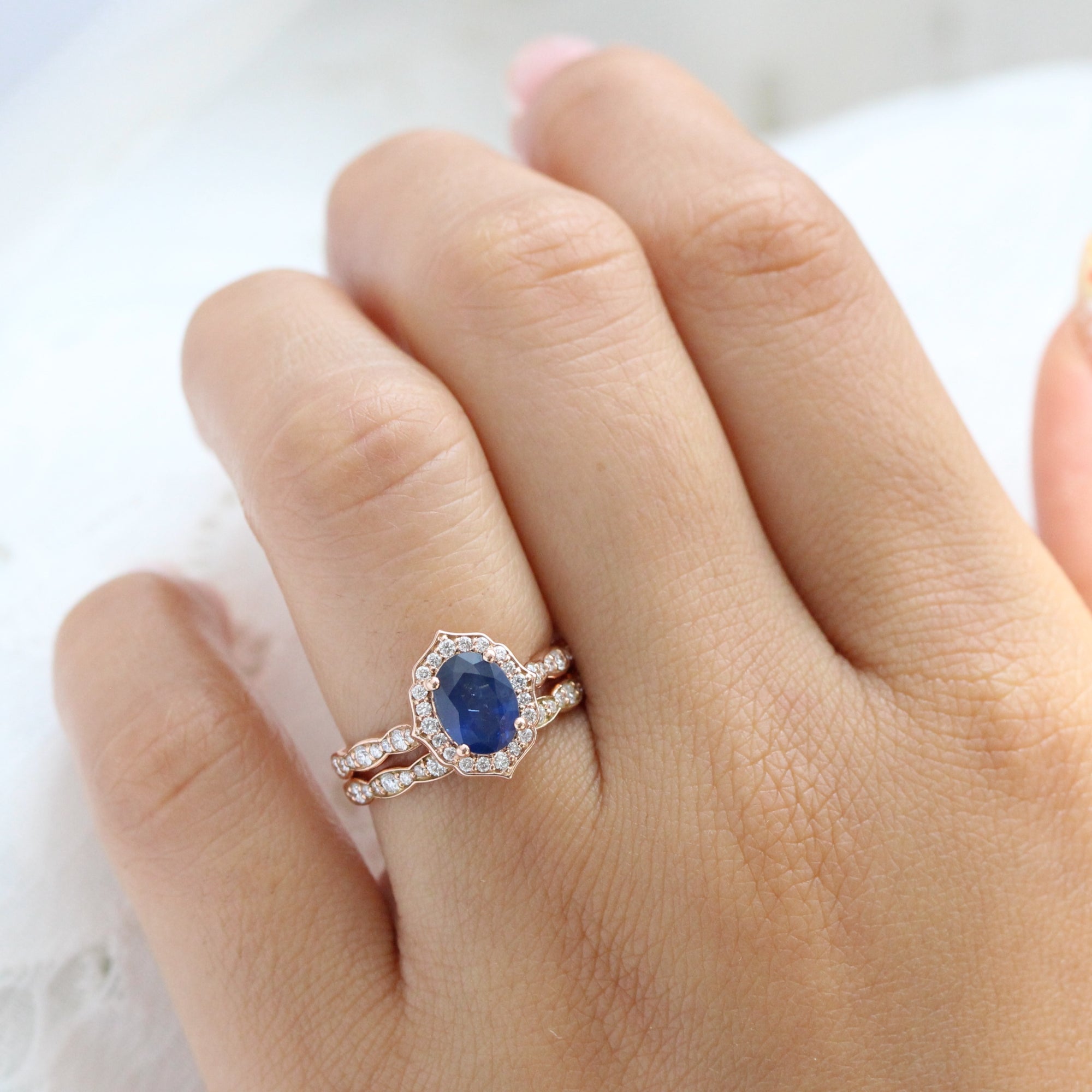The image depicts a close-up of a light-skinned, feminine hand with fingers slightly curled, resting on white fabric that resembles a wedding gown. The focus is on the ring finger, adorned with an elegant wedding set. The set features two parallel gold bands inset with diamonds. At the center of the engagement ring is an oval blue sapphire encircled by small white diamonds in a pointed casing at the top and bottom. Smaller diamonds continue down the band on either side of the central stone. The complementary band beneath the engagement ring also has matching diamonds. The background, mostly white, fades into an out-of-focus gray area in the top left corner. The detailed photograph is a square format, representing realism and product photography.